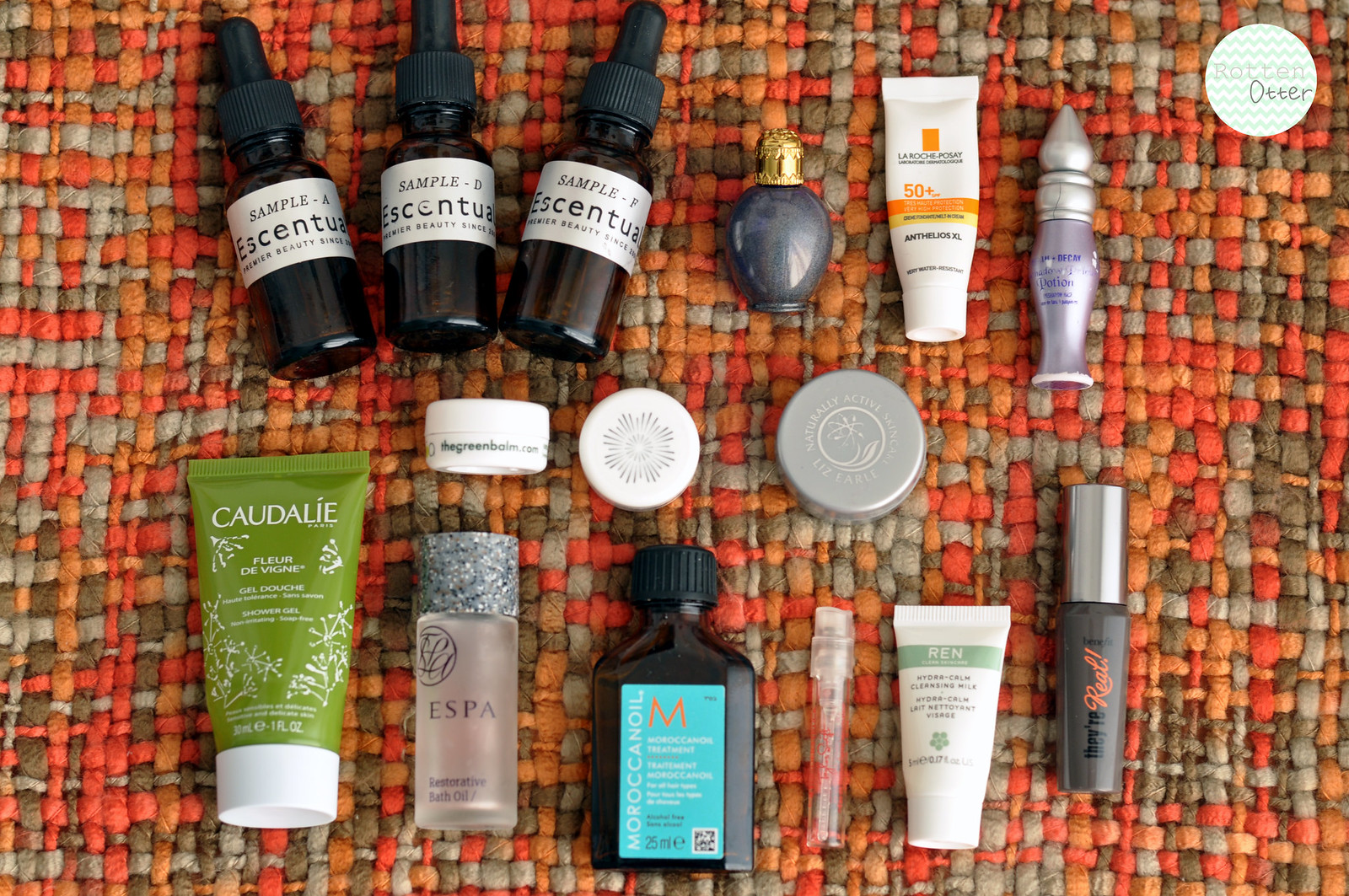This photograph showcases an assorted collection of beauty products meticulously arranged against a white background. In the top left corner, there are multiple sample scent bottles neatly lined up. Each bottle is clearly labeled with the word "sample" in small black text, followed by the brand name "Scentist" beneath it. These sample bottles feature a minimalistic design with black text on a white background.

Moving to the top right corner, a variety of other beauty bottles are displayed. Notably, there is an elegant black perfume bottle capped with a golden top, exuding a sense of luxury. Next to it, there appears to be a lotion bottle distinguished by orange accents. Another striking bottle in this section resembles a perfume container, boasting a heart-shaped top and a vibrant purple base, adding a whimsical charm.

In the bottom right area, an eyeliner with a silver cap and a black base is positioned prominently. Despite having some text on it, the writing is illegible from the angle of the photograph.

Further down, additional bottles are scattered. One of them, presumably a lotion bottle, can be identified by its green stripe, although the brand name remains unclear. Situated in the bottom left corner, a bottle branded "Kaldail" catches the eye. This bottle is unique with its green and white color scheme, where the cap is white and the base transitions to green, albeit positioned upside down.

Overall, this detailed array highlights an eclectic mix of beauty products, each with distinct designs and colors, creating a visually appealing collection.